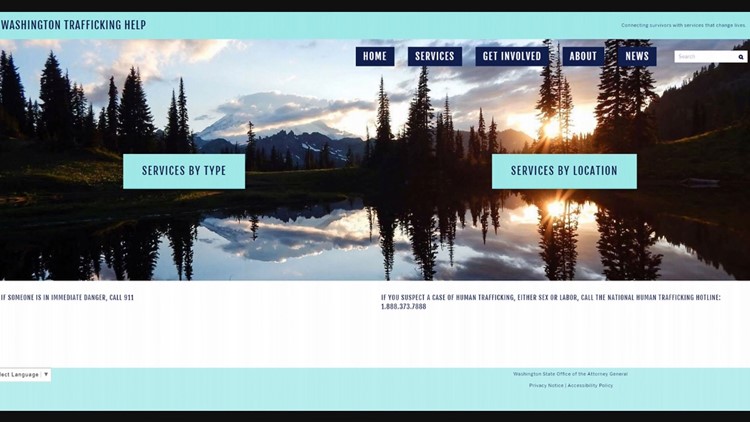Set against a white background, this vivid image captures a picturesque mountainous landscape during sunset. The sun is seen dipping behind the mountains on the right side of the scene, casting a radiant palette of blues, grays, and golds across the sky and reflecting beautifully on a tranquil lake that stretches from the bottom of the photo. Majestic pine trees are densely clustered on a hill to the left, with more appearing in the distance on the upper right.

In the upper left corner of the image, the text "Washington Trafficking Help" is prominently displayed. Two blue action buttons are situated below this text: one labeled "Services by Type" and the other "Services by Location." 

Beneath the image, the text advises: "If someone is in immediate danger, call 911. If you suspect a case of human trafficking, either sex or labor, call the National Human Trafficking Hotline." Further information can be found by visiting www.FEMA.gov.